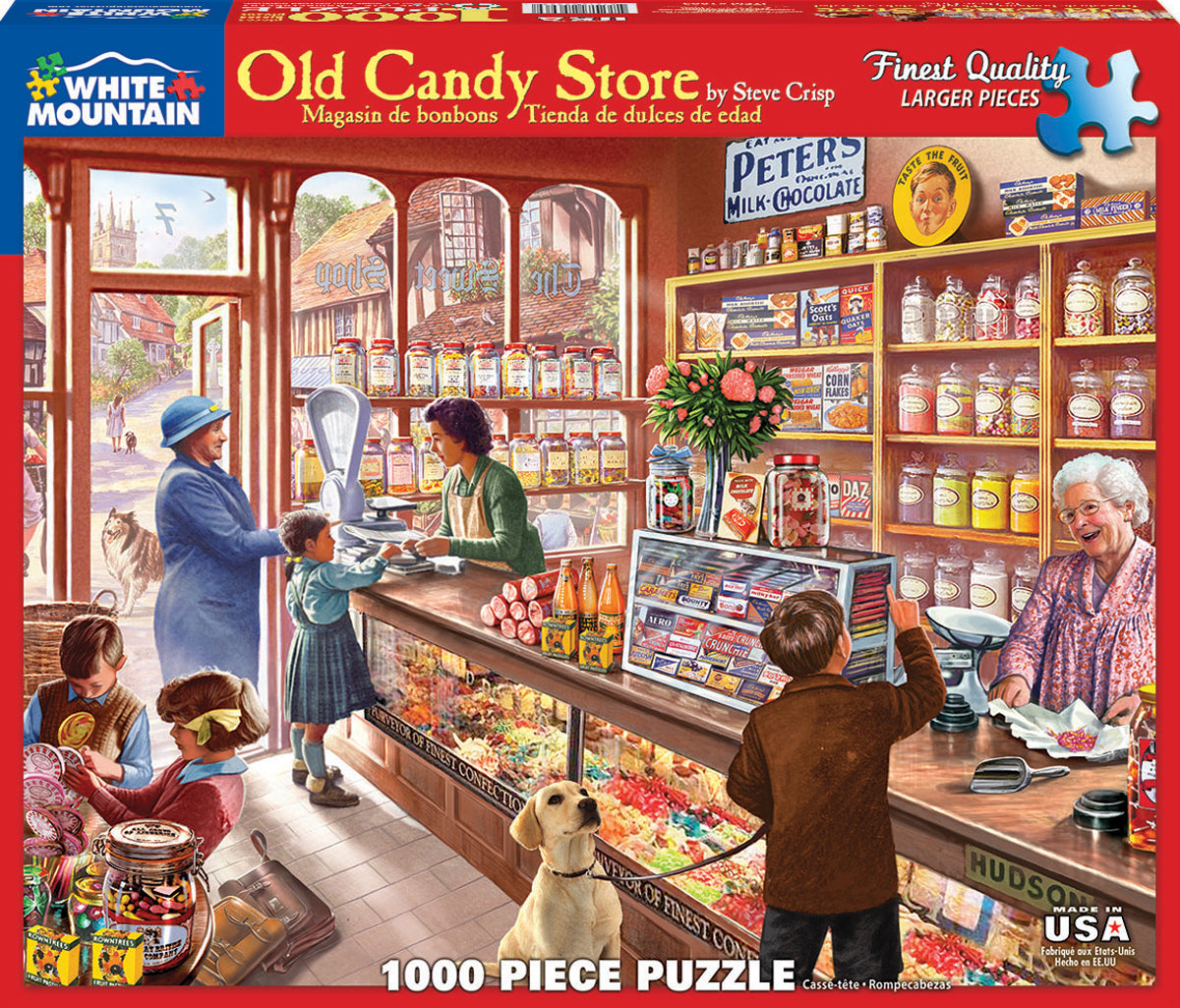The front of this puzzle box is bordered in red and prominently features a quaint old-fashioned candy store. In the top left corner, a small blue section displays the "White Mountain" logo in white letters. The main title, "Old Candy Store" written in yellow, is accompanied by a description in Spanish. The artist's name, "Steve Crisp," is noted near the title. Emphasizing its quality, the box states "finest quality larger pieces" in white letters along with an illustrated blue puzzle piece. At the bottom, the box indicates that it is a thousand-piece puzzle with the text "1000 piece puzzle" in white.

The central image on the box depicts an engaging scene within the candy store. An older woman with white hair and glasses, smiling warmly, stands behind a counter assisting a young boy and his yellow Labrador, who are choosing candy together. On the right side of the counter, another saleswoman is seen weighing candy for a small girl accompanied by her mother. Scattered throughout the store, other children are visible, some examining a display of large lollipops. This detailed and nostalgic artwork captures the lively atmosphere of the candy store, filled with colorful candies and cheerful interactions.